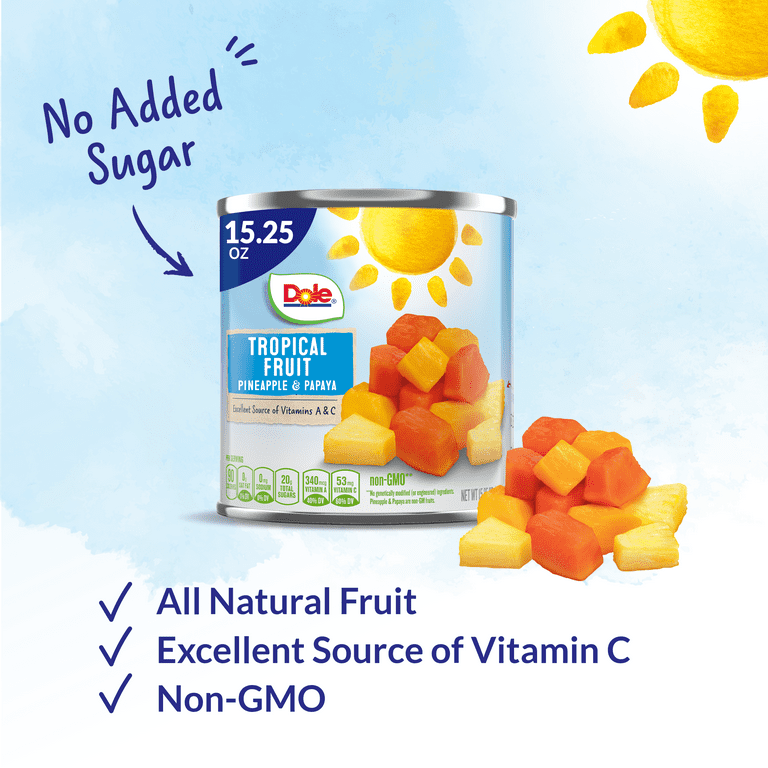The advertisement showcases a can of Dole Tropical Fruit Mix—specifically pineapple and papaya—highlighted against a backdrop of a clear blue sky adorned with fluffy white clouds and a radiant yellow sun. At the top, bold blue lettering proclaims "No Added Sugar," with three small blue lines emanating from the text, directing attention to the can. The can prominently reads "15.25 ounces, Dole Tropical Fruit, Pineapple and Papaya," and emphasizes its status as an "Excellent Source of Vitamins A and C." Below, a nutritional label subtly confirms the product is "non-GMO."

In the bottom section of the ad, additional blue captions feature checkmarks next to key selling points: "All Natural Fruit," "Excellent Source of Vitamin C," and "Non-GMO." Complementing the textual information, a vibrant pile of mixed fruit—showcasing hues of yellow, pink, and orange—sits next to the can, visually mirroring the fruit imagery depicted on the can’s label, which also includes the iconic Dole logo with a yellow sun.